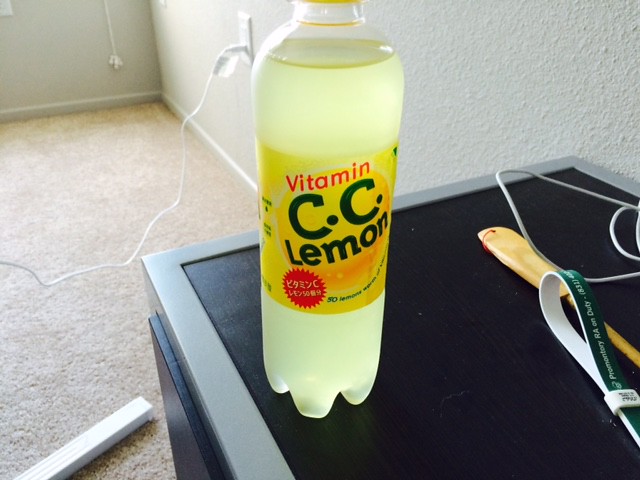This color photograph, taken indoors, features a tall, clear bottle of soft drink labeled "Vitamin C.C. Lemon." The bottle contains a light yellow liquid and has a yellow cap that is partially visible. The label around the middle of the bottle is bright yellow, featuring green text for "C.C. Lemon" and red text for "Vitamin," with additional non-English characters that could be Japanese, Korean, or Chinese. The bottle is placed on a rectangular black surface with a silver border, which is likely part of an entertainment center or mini-fridge. The scene includes several objects on and near this surface: a white cable coming from a mid-wall outlet and extending bent across the floor, a lime-green and grey wrist strap, wooden sticks, and a small wooden implement with a red thread. The room has light beige carpeting, and the walls are white and textured. The area appears sparsely furnished, suggesting someone may be in the process of moving in or out.